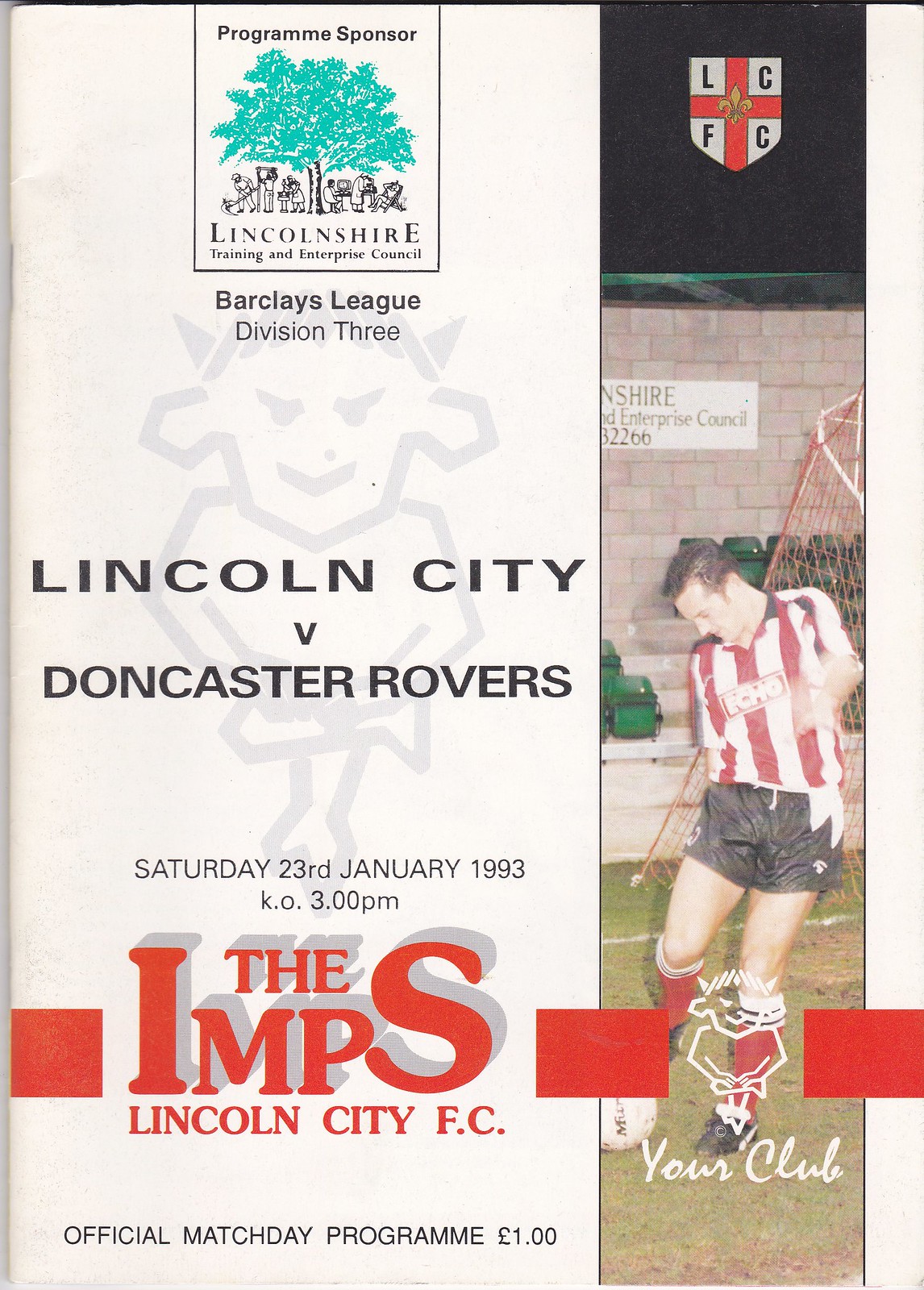The image showcases the front cover of an official match day program for a soccer game. The vertically aligned rectangular design prominently displays the event details and graphics. At the top, there's a small section labeled "Program Sponsor," featuring a green tree icon followed by the text "Lincolnshire Training and Enterprise Council." Below that, in black text, it states "Barclays League Division 3," leading to the match details: "Lincoln City vs. Doncaster Rovers," scheduled for "Saturday, 23rd January 1993," with a kickoff time of "3 PM."

Central to the layout, a bold red strip reads "The Imps, Lincoln City F.C.," with "The" positioned above "IMPs" in a large font. At the very bottom, in smaller black text, it declares "Official Match Day Program, One Pound."

On the right-hand side of the cover, a narrow vertical section features a badge with a red cross and the letters "L C F C" in white squares around it. Below the badge, there is an action photo of a soccer player in a red and white vertical striped jersey, black shorts, red socks, and black cleats, captured mid-kick. Underneath his feet, the grass is marked with the text "Youth Club." The overall design and content suggest this program was intended for attendees of the Lincoln City vs. Doncaster Rovers match, serving both as a souvenir and informative guide for the event. The color scheme includes prominent reds, blacks, and whites, with additional accent colors like green and blue.